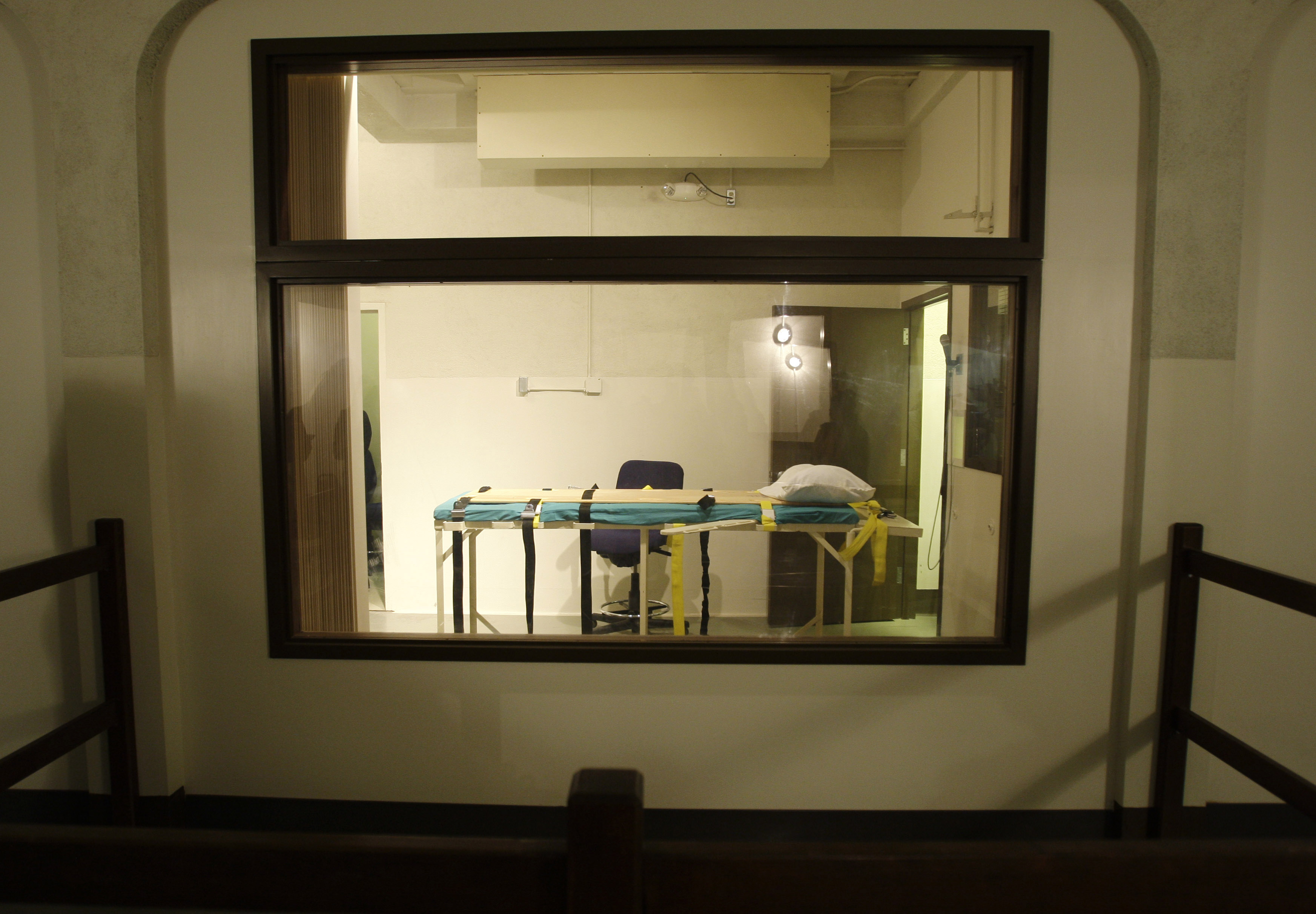This image depicts the stark setting of an execution chamber viewed from the witness room. The vantage point shows wooden benches with separations, likely where witnesses would sit, facing a large double-panel window, each pane framed in dark brown wood. The upper pane is narrower, separated from the taller bottom pane by a horizontal frame. 

Through these rectangular windows, the sterile room within comes into view, characterized by its stark white walls. Centrally positioned is a gurney used for lethal injections, identifiable by its blue mattress and white pillow on the right. The gurney features a tan backboard fitted with multiple black and yellow straps, designed to secure the individual. Beneath the gurney, a teal cover adds a splash of color, and the entire setup is mounted on a stand. 

Flanking the gurney are doorways on both the left and right sides, suggesting additional access points possibly used by staff. A blue office chair sits behind the gurney, unoccupied at this moment, enhancing the room’s clinical and somber atmosphere. A reflection in the window indicates the absence of people in both rooms.